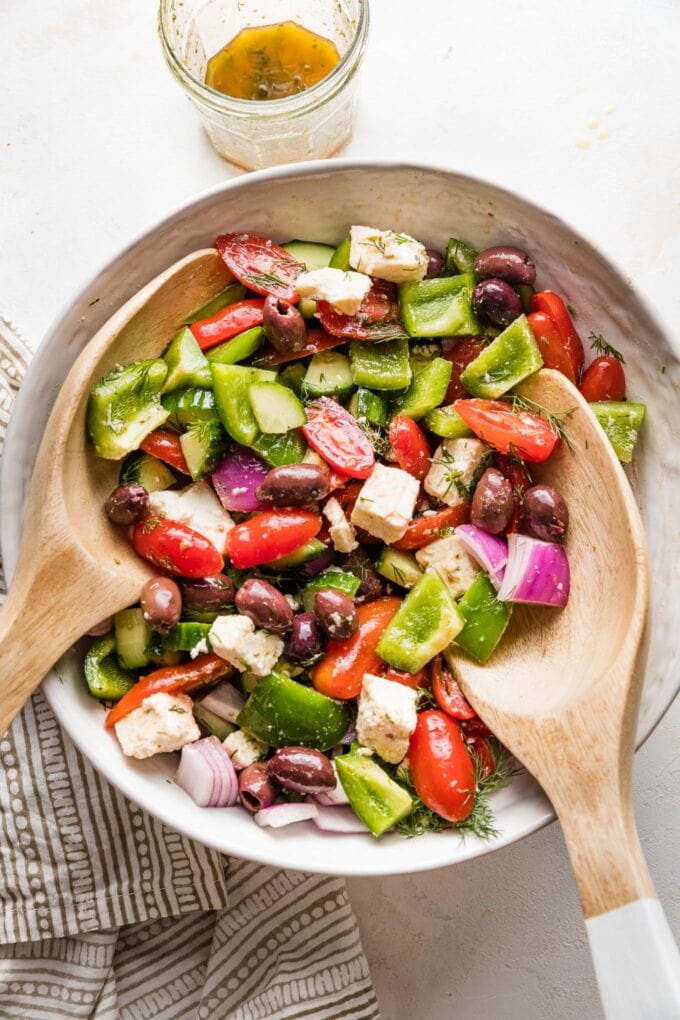This image captures a top-down view of a vibrant and colorful salad presented in a white, textured ceramic bowl. The salad is a mix of cubed chicken, green and red bell peppers, cherry tomatoes, purple onion, kalamata olives, and either brown or black beans, all garnished with fresh herbs. Additionally, there's a sprinkling of seasoning throughout the salad. Two large wooden spoons, one of which has a white handle, are placed inside the bowl, partially obscured by the ingredients. The bowl rests on a white tea towel adorned with a brown design that includes stripes, dots, and rectangles with horizontal lines. To the side, there is a clear glass filled with an orangish-yellow liquid, likely the salad dressing, all set on a clean white countertop.